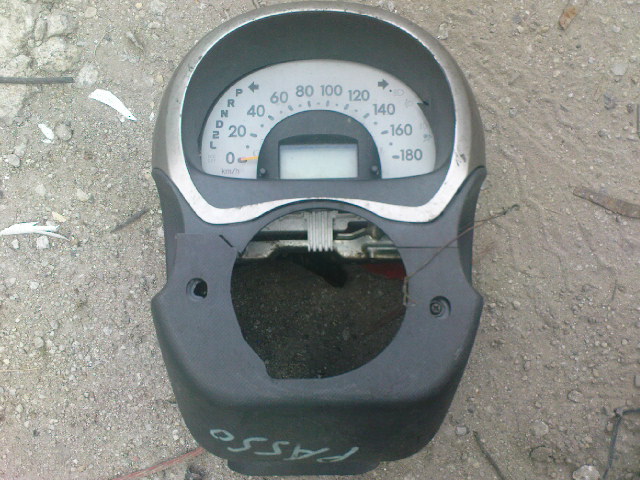This photograph features a disassembled automotive steering column, positioned on a patch of loose, brown dirt. The primarily black column is adorned with a silver accent around its top. Prominently displayed in a semicircular arrangement on the left side, the gear shift indicators read: Park (P), Reverse (R), Neutral (N), Drive (D), Second gear (2), and Low gear (L). Adjacent to this, the speedometer extends from 0 to 180 miles per hour. Notably, beneath the speedometer, there is a smaller odometer for tracking mileage. The base of the steering column features the brand marking "PASSO." The entire assembly appears detached from its original vehicle, discarded and resting on the ground.